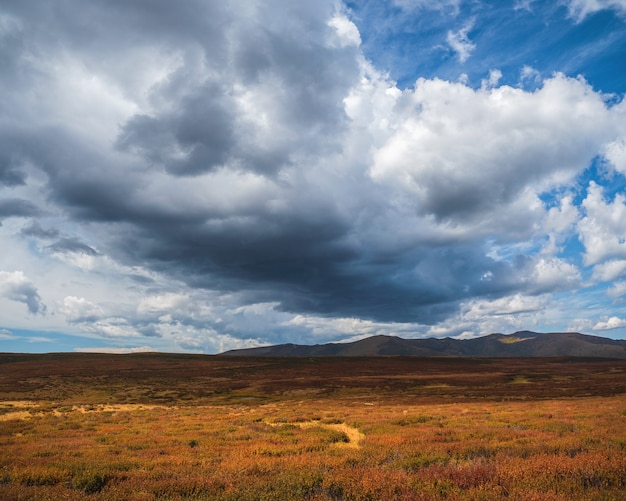This horizontal rectangular image captures a vast desert or Midwest landscape scene in the fall, dominated by a sprawling sky that occupies over half of the frame. The foreground is a mix of tan, brown, and sparse green ground cover, indicating dead or dry vegetation, with patches that appear to be sand or clear dirt. A feature runs through the middle that could be either a road or a dry riverbed, adding depth to the expansive flat terrain. The background reveals a range of shadowed mountains stretching almost the entire width of the image, with some areas highlighted by a yellowish tint. Some hills are dotted with trees with green leaves, though they are less prominent. The sky above is a dramatic display, featuring a substantial cloud formation obscuring much of the mountains, with heavier gray clouds concentrated in the middle and patches of blue sky visible both above and below the clouds. This composition emphasizes the expansive and open nature of the landscape, framed by the overarching presence of the sky.